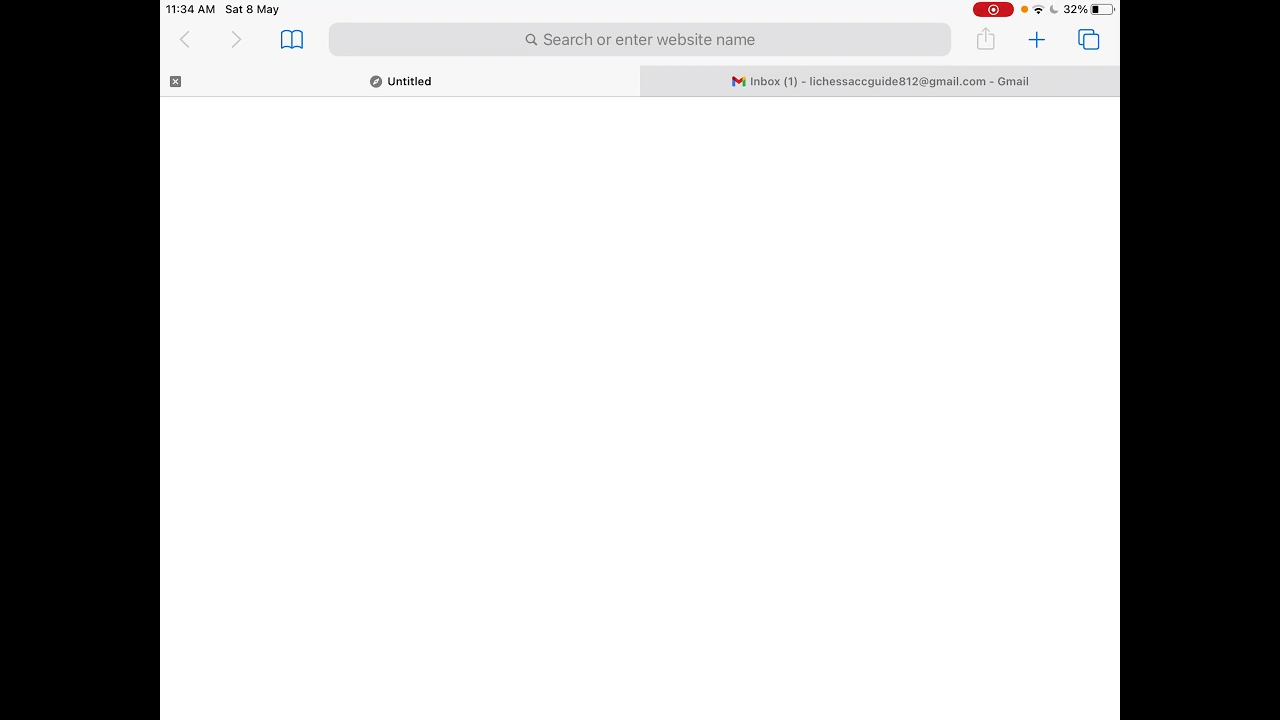The image showcases the interface of a web browser displaying a new and untitled tab. The page is blank, indicating that the settings have been configured to open an empty tab each time a new one is initiated by clicking the plus sign. On both the left and right sides of the screen, there are thick vertical black lines, framing the visible browser area.

In the upper left-hand corner, the current time is displayed as "11:34 AM" in black font. Adjacent to the time, to the right, the date is shown as "Sat 8 May," indicating it's Saturday, May 8th. On the upper right-hand side of the screen, there is a prominent red button that appears to signify live recording, accompanied by an icon indicating the device's battery level, which is at 32%.

Below these elements sits the search bar, with the placeholder text "Search or enter website name." Additionally, one of the active tabs visible is labeled "Gmail inbox," suggesting that the user's email account is open in another tab.